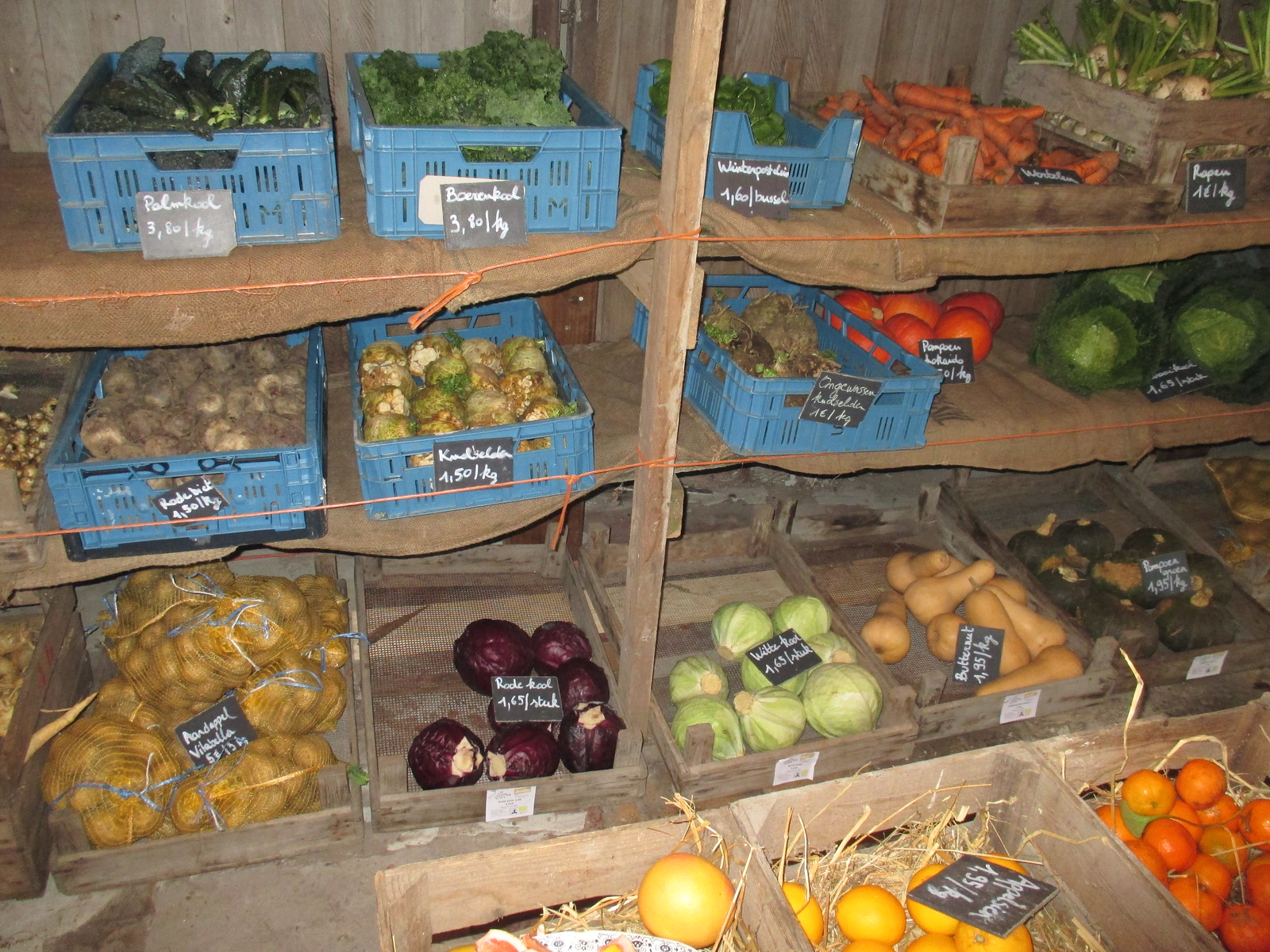The photograph depicts an impeccably organized display, possibly from a farmer's market or farm shop, featuring three sturdy wooden shelves laden with an assortment of vegetables housed in both blue plastic and brown wooden containers. The top shelf showcases cucumbers and broccoli on the left, with carrots occupying the right. The middle shelf displays lettuce and tomatoes, while the bottom shelf hosts various types of squash, turnips, and potatoes. The containers are clearly marked with handwritten signs indicating the types of vegetables and their respective prices per weight or item, though the details are somewhat difficult to read. In front of the shelves, some wooden containers filled with fruits like oranges rest on the ground, accompanied by yellow-orange rope draped across the shelves, adding a splash of color. Hay is visible beneath some of the produce, enhancing the rustic and authentic farm ambiance. The setting appears to be well-lit, suggesting it might be an outdoor market space.